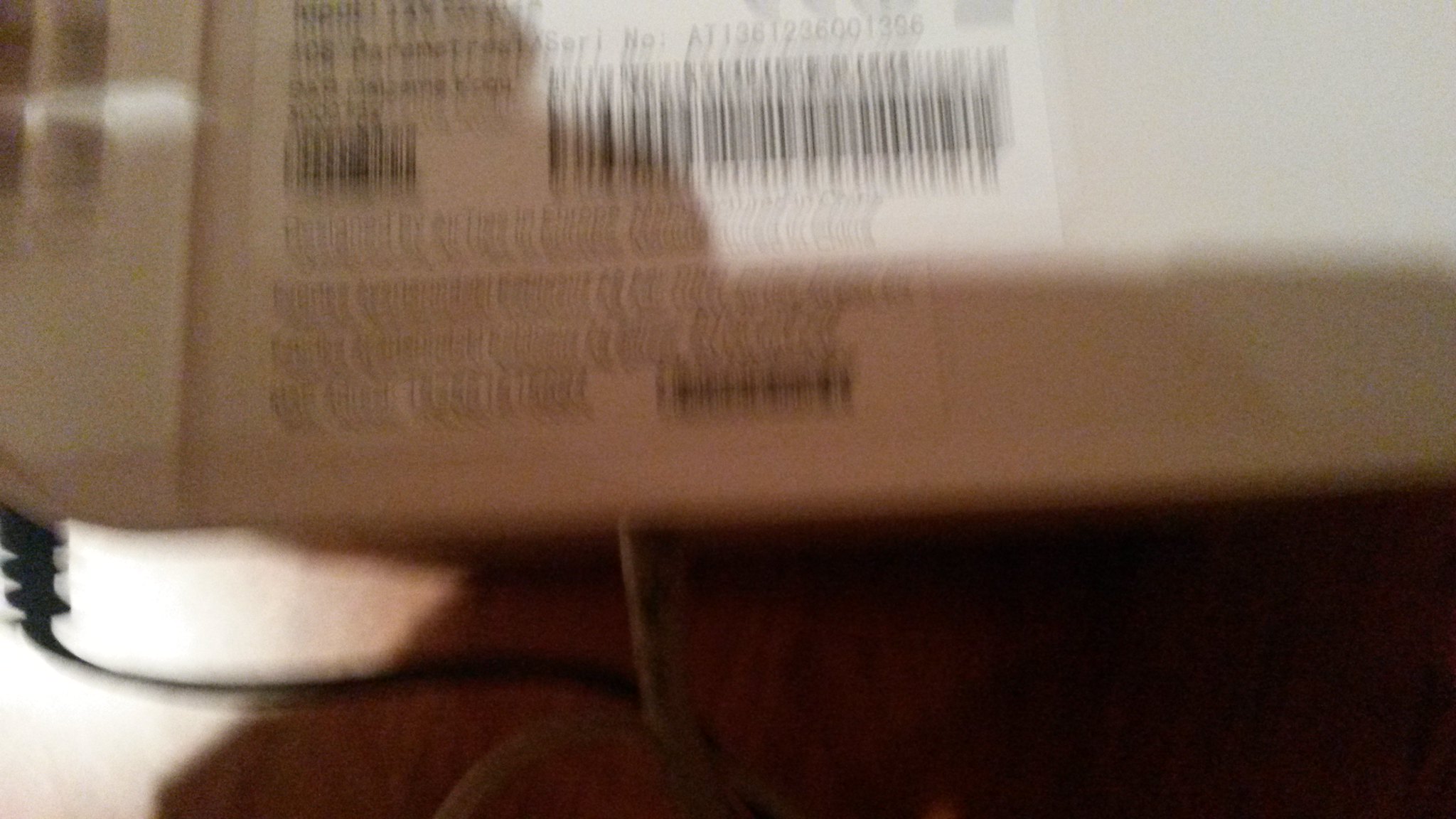The image predominantly features a shadow cast over an object, creating a boxed-in effect with white surrounding most of the frame. At the very bottom, there is a distinct black shadow. In the top left corner, the background is primarily white with some wavering text and a blurry, out-of-focus barcode. Additionally, at the bottom left corner, a cable is visibly plugged into the object, with some text nearby, although it's difficult to decipher the specifics. Overall, the image captures an abstract, partially obscured scene with elements of text and technology hinting at a larger context.